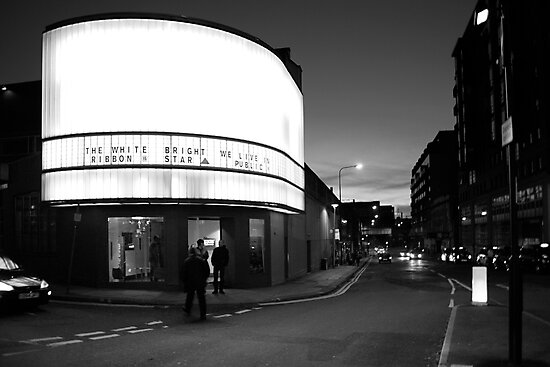The black-and-white photograph, taken outdoors at nighttime and measuring approximately four by three inches, captures a city street corner with several notable details. On the left-hand side, a prominent building features a large, curved marquee sign that is nearly twice the height of the building itself. The marquee displays the text: "The White Ribbon, Bright Star. We live in public." Below the brightly lit marquee, a doorway reveals a few people standing inside. In front of the building, a car is parked on the street. The right-hand side of the image shows the street stretching away with tall buildings extending up to the top of the photo. The scene is set against a gray, cloudy night sky, creating a moody atmosphere typical of a quiet city night.